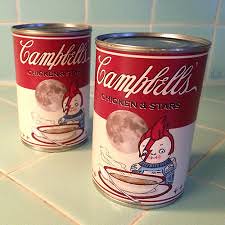The image showcases two identical cans of Campbell's Chicken and Stars soup, arranged on a light blue ceramic-tiled countertop. The same tiles extend up the wall, forming a cohesive backsplash. Each can, adorned in Campbell's iconic red and white, features a whimsical illustration: A fanciful moon and an animated young boy in a space suit with a lightning bolt design on his face and spiky red hair. The boy is depicted enjoying soup from an exaggeratedly oversized bowl. Both cans are precisely positioned at the same angle, emphasizing their identical nature.